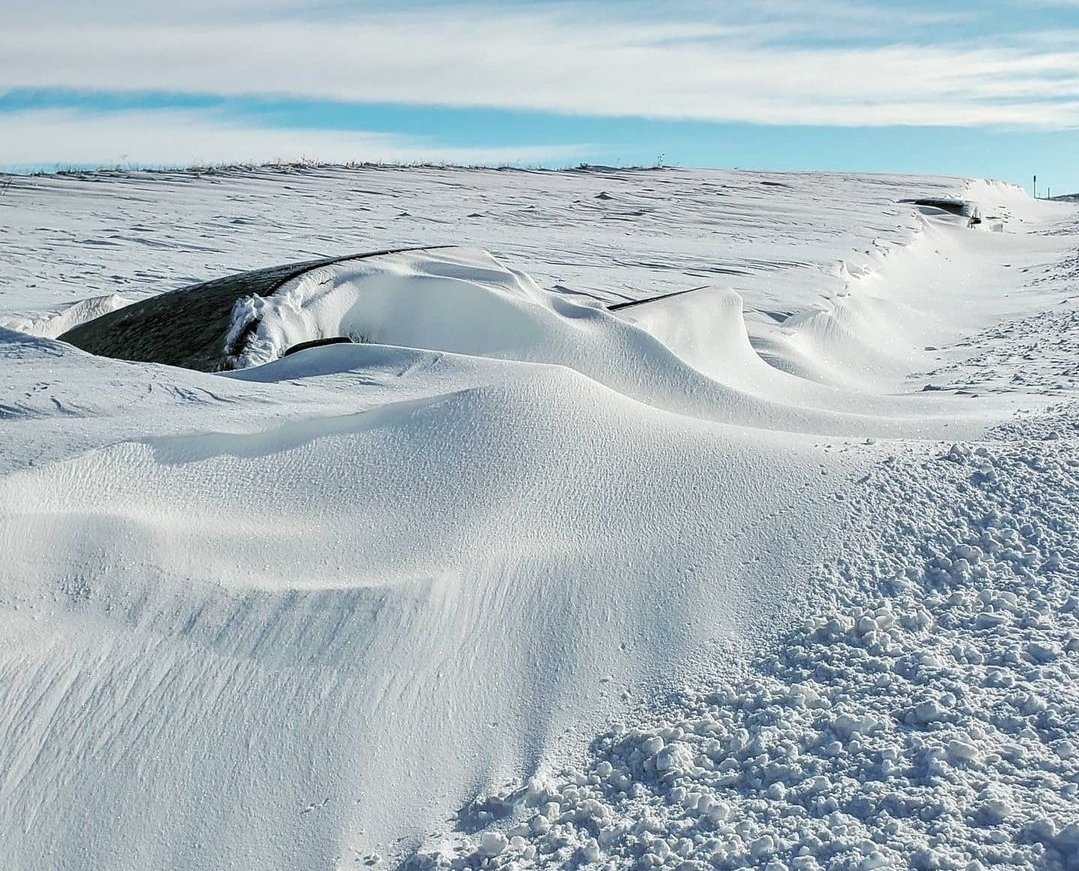This photorealistic image captures a vast snowy landscape reminiscent of an arctic tundra, possibly Antarctica. Taken from a higher vantage point—either a drone or someone standing on a snow-laden elevation—the scene is dominated by expansive snow drifts and large mounds of snow that resemble sand dunes, lending a surreal "beach meets mountain" effect. The snow appears both smooth and rugged, with some areas bearing the texture of wind-polished drifts while other sections look disturbed, as if traversed by people, animals, or a snowcat. These disturbed areas feature irregular, cotton ball-like formations amidst the otherwise smooth terrain. In the distance, traces of vegetation peek through the snow cover, and a solitary telephone or electric pole stands off to the right, hinting at the fringes of civilization. The sky overhead is a bright blue, dotted with wispy white clouds, reinforcing the stark and cold beauty of this remote, snowy expanse.